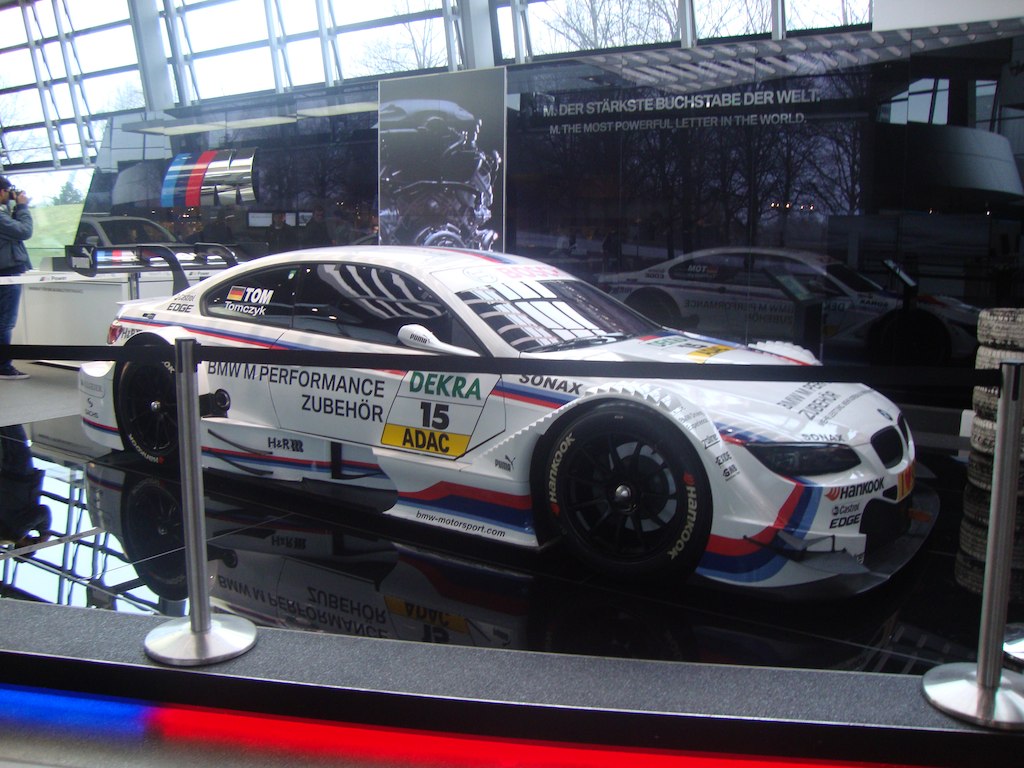This image captures a white BMW racing car prominently displayed in an exhibition showroom in Germany. The car, which appears to be mid-pit stop, is adorned with red and blue stripes and sports black racing tires. Notable markings include "15" in black on the side, with "Dekra" in green above the number and "ADAC" in yellow below it. The words "BMW M Performance Zubehör" are also visible on the side, along with "Sonax" above the front wheel well. 

The reflective black floor enhances the car's striking appearance, mirroring its details with remarkable clarity. In the background, a glass wall reveals outdoor trees, and the top part displays windows, offering a glimpse of the exterior. A cordoned-off area with stanchions and a counter in the left middle ground are visible, adding to the exhibition setting. A single person can be seen on the far left, seemingly taking a photo of another exhibit. Above the car is German text reading "M der Stärkste Buchstabe der Welt," which adds to the authenticity of the German locale. The overall ambiance is one of a meticulous and prestigiously arranged exhibition hall, showcasing the sleek and sporty BMW amidst a modern, reflective setting.